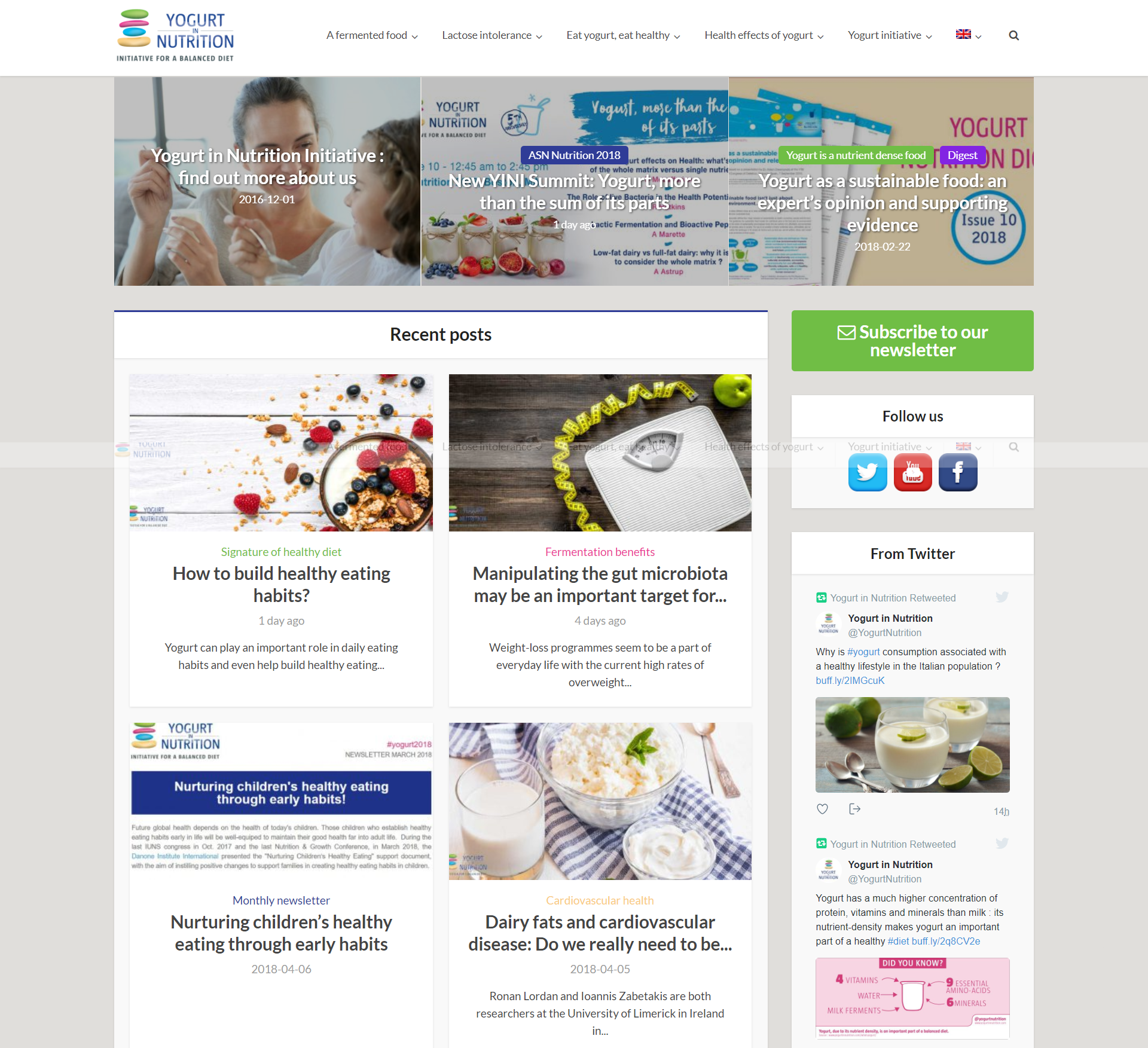Certainly! Here is a cleaned-up and detailed caption for the image:

---

The image depicts a webpage for a yogurt and nutrition initiative aimed at promoting a balanced diet. At the top left of the website, the logo features the words "Yogurt and Nutrition" stacked in blue text, with "Initiative for a Balanced Diet" written in black underneath. An icon made up of deconstructed shapes in green, red, blue, and yellow is prominently displayed. 

To the right of the logo, the headers of the page are listed in gray text: "A Fermented Food," "Lactose Intolerance," "Eat Yogurt, Eat Healthy," "Health Effects," and "Yogurt Initiative." Further to the right, a UK flag icon resembling a briefcase is displayed, accompanied by a drop-down arrow and a magnifying glass icon.

The top left section of the page features banners. The uppermost banner shows an image of a mother and young child with the text "Yogurt and Nutrition Initiative" and "Find More About Us" written in white. To the right of this, another banner states "YINI Yogurt Line" in white on a slightly faded background.

In the background, a home page or benefits page is visible. On the right side, a section reads "Yogurt is a Sustainable Food: Experts' Opinions and Supporting Evidence," displayed in white text on a beige backdrop. Below, a "Recent Posts" section lists four articles in black text, each accompanied by an image. The articles are titled: 

1. "Healthy Eating Habits: The Role of Manipulating Gut Bacteria"
2. "Talk it Forward..."
3. "Nurturing Child's Healthy Eating Habits"
4. "Dietary Fats and Cardiovascular Disease: Do We Really Need to..."

The overall design is clean and informational, focusing on various aspects of yogurt consumption and nutrition.

---

This detailed caption provides a comprehensive overview of the webpage's content and layout.